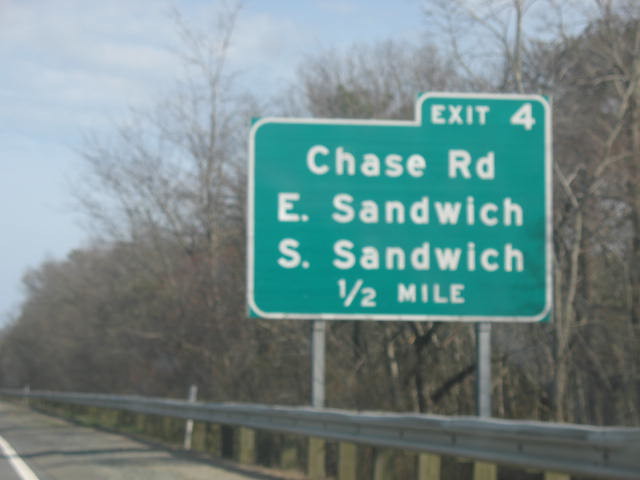The photograph captures a winter scene along a highway, marked by a silver guardrail that stretches from the bottom right to nearly the center left. Dominating the image is a green road sign with white text indicating "Exit 4, Chase Road, East Sandwich, South Sandwich, 1 1⁄2 mile," shaped like a rectangular file folder with a tab at the top right. The surroundings are characterized by dormant trees with bare brown branches, casting shadows on the left side of the road. The sky above is a mix of blue and cloudy, suggesting a partly cloudy day. A small section of the white painted road line is visible, enhancing the roadside view from a vehicle’s perspective.